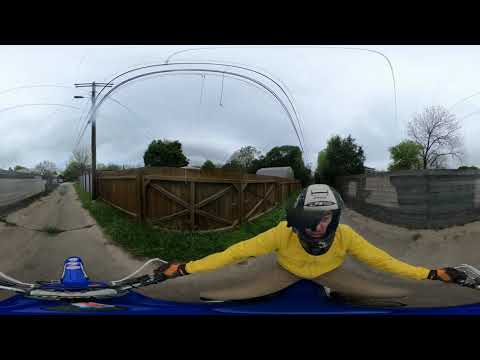This dynamic outdoor photograph, taken with a fisheye or 360-degree lens, features a person riding a blue dirt bike down a narrow, sandy-colored road. The rider is clad in a vibrant yellow, long-sleeved jacket, khaki pants, and a helmet that is predominantly gray with black accents, designed for motorsport activities. The road, flanked by contrasting fences—one a curved wooden structure and the other a gray concrete barrier—appears to wind through an alley-like landscape. The sky overhead is overcast, filled with white and gray clouds, adding a moody atmosphere to the scene. In the background, a mix of trees, some lush with leaves and others bare, extends toward the horizon. Additional elements captured include power lines on poles and verdant grass alongside the road, visually connecting the scene from the curving boundaries to the stretched horizon.